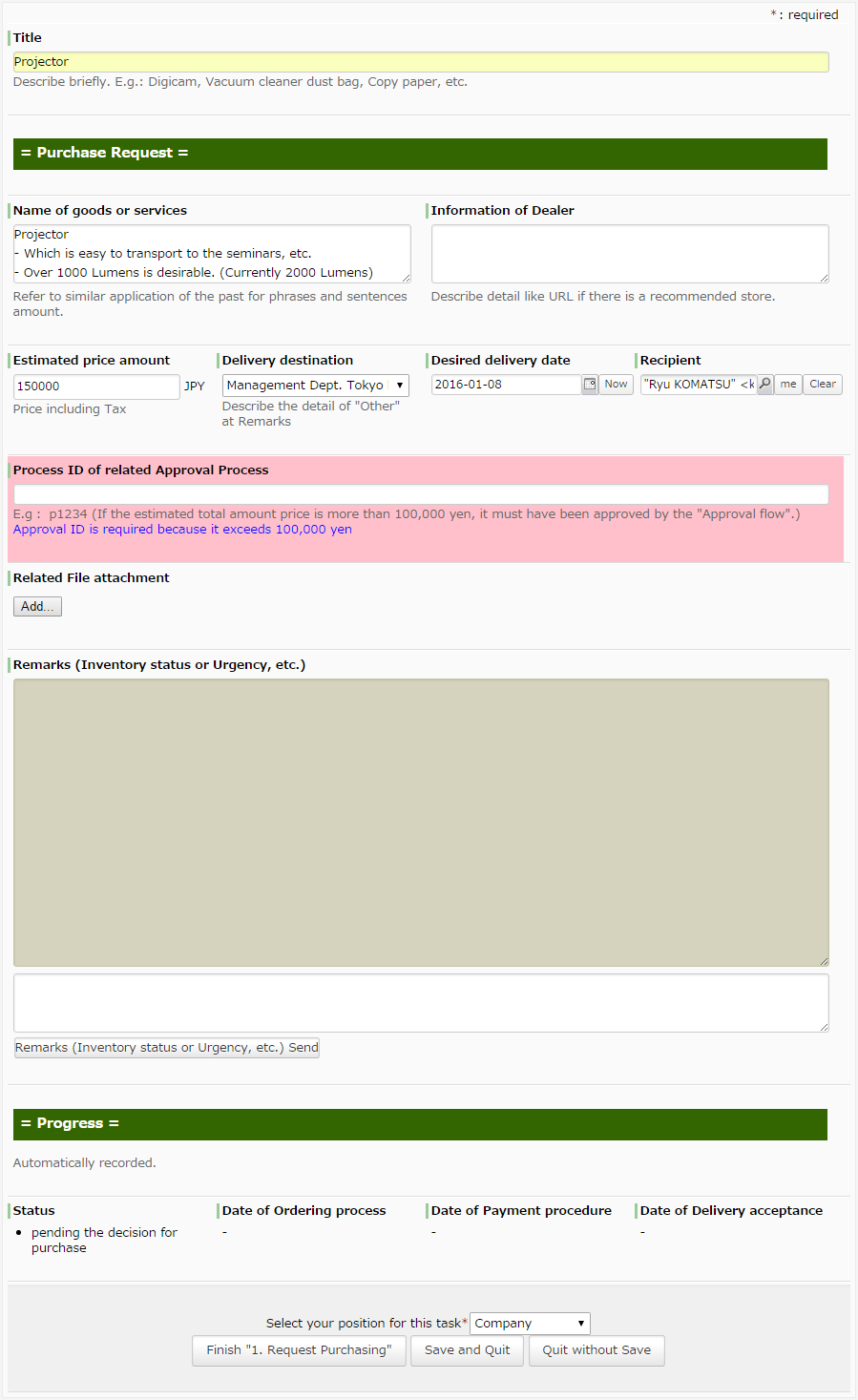This image, sourced from a website, depicts a detailed purchase request form designed for an employee to complete. 

At the top of the form, the user is asked to provide a title, where "Projector" has been typed. Below, there's an instruction to briefly describe the item, with examples such as "digicam, vacuum cleaner, dust bag, copy paper, etc." Following this is a section labeled "Purchase Request," highlighted with a green banner. 

In the "Purchase Request" section, several fields are available for input:
- **Name of Goods or Services**: "Projector, which is easy to transport to seminars, etc., and over 1,000 lumens is desirable, currently 2,000 lumens."
- **Information of Dealer**: This field remains empty.
- **Estimated Price Amount**: "$150,000."
- **Delivery Destination**: "Management Department, Tokyo."
- **Desired Delivery Date**: "2016-01-08."
- **Recipient**: "Ryu Komatsu."

Following this, there's a section for the "Process ID of Related Approval Process," which hasn't been filled out. There's also an area to attach related files, if necessary.

Further down, there's a section for additional remarks, including inventory status or urgency, but it is currently blank.

At the bottom of the form, there's a "Progress" section where statuses such as date of ordering, payment procedure, and delivery acceptance are automatically recorded. Lastly, the user can select their position for this task, marked as "Company."

To finalize the form, users have three options: "Finish," "Request Purchasing," "Save and Quit," and "Quit Without Save."